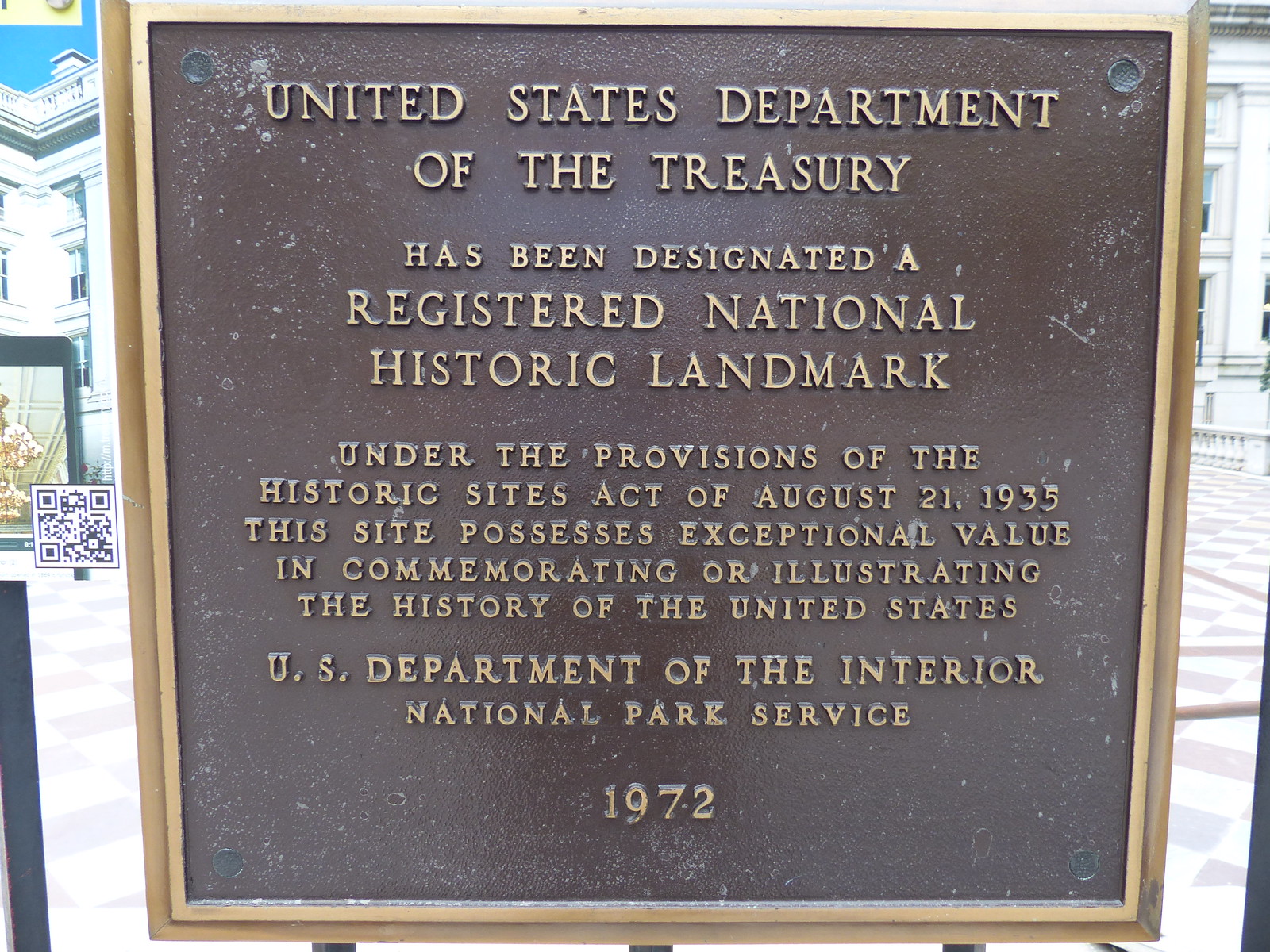The image prominently features a large, bronze historical placard framed by a brassy gold border. The center of the placard, displayed in a square shape, has a brown background with gold text. The heading reads "United States Department of the Treasury" and it states that the site "has been designated a registered National Historic Landmark under the provisions of the Historic Sites Act of August 21, 1935." The placard further notes that the site "possesses exceptional value in commemorating or illustrating the history of the United States" and is recognized by the "U.S. Department of the Interior National Park Service." At the bottom, the date "1972" is inscribed. To the left of the placard, there is a QR code that likely provides more information. In the background, white Greco-Roman revival architecture government buildings, along with a plaza featuring white and red tiling, are visible, suggesting that the location might be in Washington, D.C.